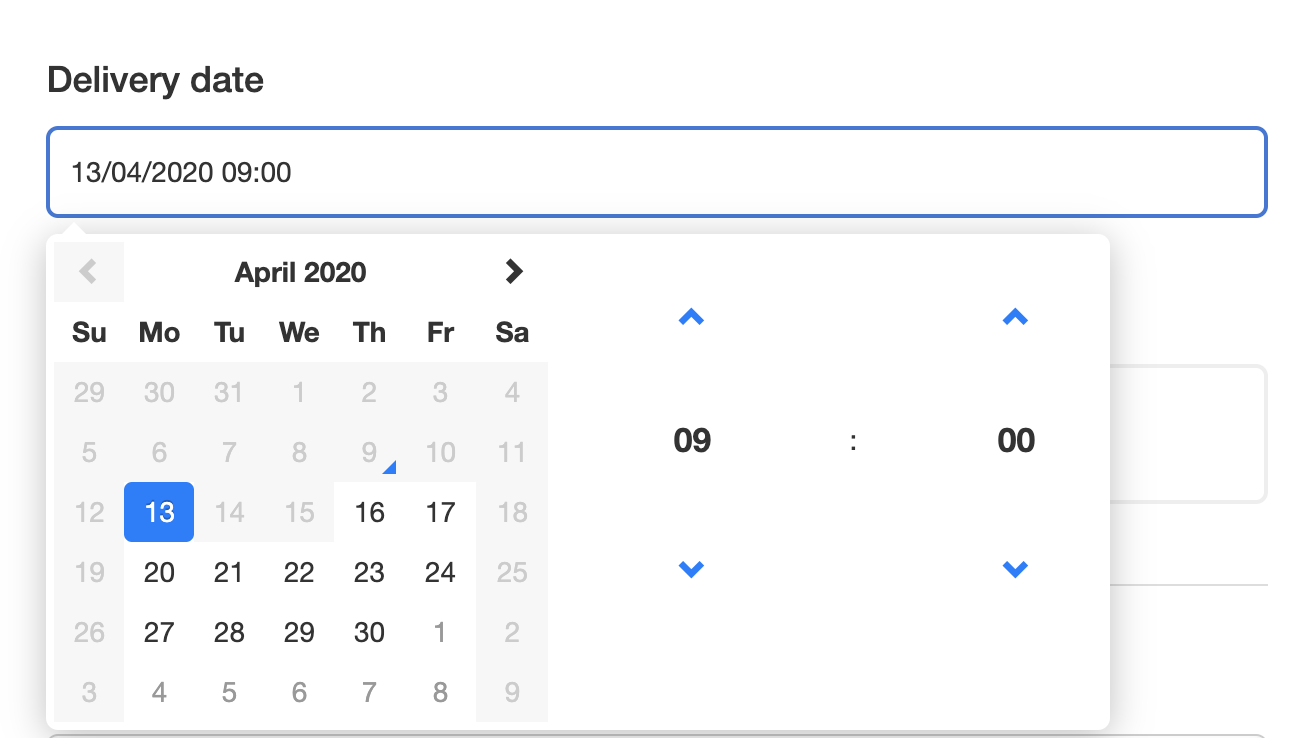In the image, the delivery date is displayed in the upper left corner. There is a horizontal bar extending the full width of the screen, containing the date "13/04/2020" at "09:00". This bar is outlined in blue, with a white interior. Below it, a calendar is shown with "April 2020" prominently labeled at the top. The date "Monday, 13th" is highlighted with a blue square and white text reading "13." 

Dates from "14" to "19" as well as those for Saturday and Sunday are all shown with a gray background and gray numbers. Dates from the "20th to the 30th" are shown in black text on white backgrounds. On the right side of the calendar, there is a distinctive square displaying the number "9" with a blue arrow pointing upwards above it and another blue arrow pointing downwards below it. 

Additionally, there is a side section marked "00" with similar blue arrows above and below the numbers. This whole calendar pop-down obscures some fields below it, which are outlined in gray but currently not visible due to the drop-down calendar. 

The color scheme of the image primarily features black, white, blue, and gray elements.